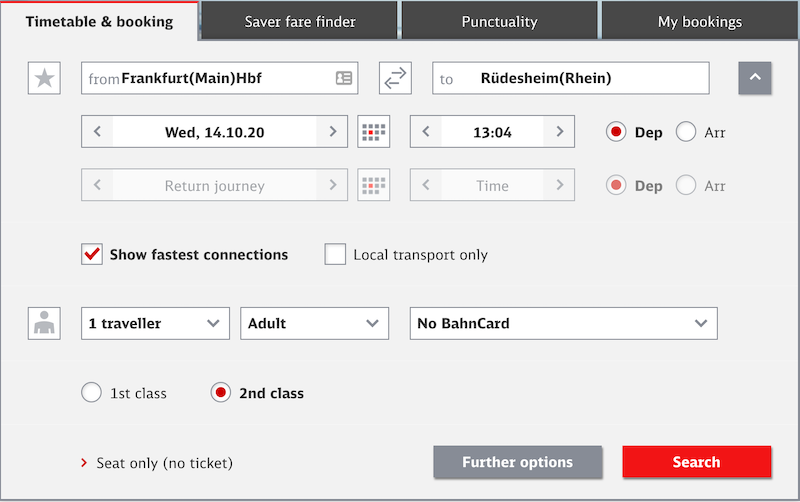"Screenshot of a transportation booking site. The specific mode of transportation is not identified, and the available tabs at the top include 'Timetable and Booking,' 'Sabre and Farefinder,' 'Punctuality,' and 'My Bookings.' The highlighted tab is 'Timetable and Booking.' The journey is scheduled from Frankfurt to Rüdesheim on October 14th, 2020, departing at 13:04 (1:04 PM). It is a one-way trip for a single adult traveler. The 'Show fastest connections' option is selected, while the 'Local transport only' option remains unchecked. The traveler does not possess a BahnCard."